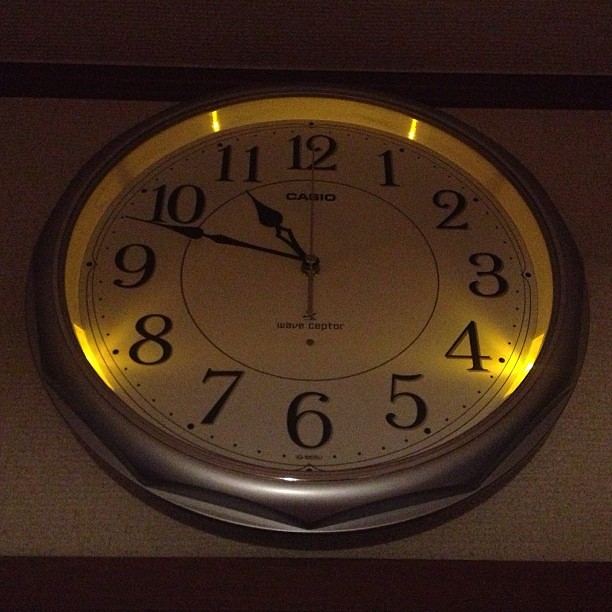In the center of the image, there is a dimly lit, round Casio clock with a silver metal frame and a white face. The clock is affixed to a wall that appears to be made of cork or covered in a light brown textured wallpaper, framed by a dark-colored border, either brown or black. The clock features black numbers from 1 to 12, and the black hands are ornate with spade-shaped tips. There is a gold second hand. The Casio brand name is positioned at the top of the clock face under the number 12, while "Wave Ceptor" is written above the number 6, accompanied by a small dot. The minute hand is 2 dots away from 10, indicating the time is approximately 10:48. The clock appears to have internal lighting that illuminates parts of the numbers from the side, adding a subtle glow to the face.